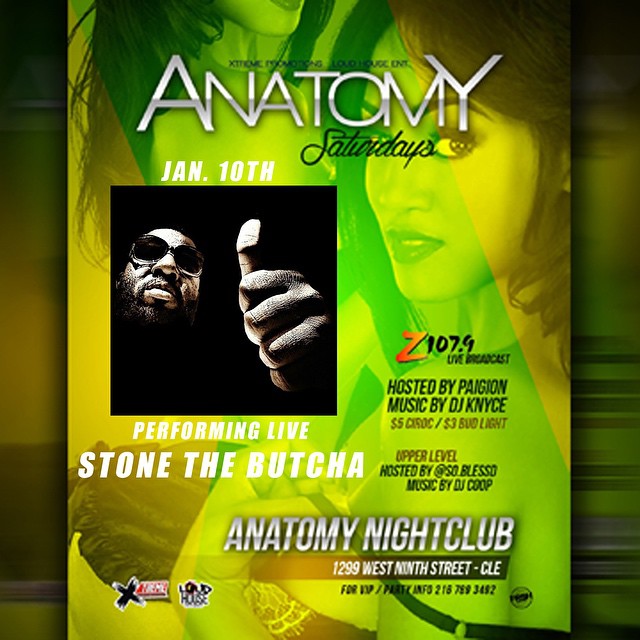The advertisement features a visually striking layout with a green and yellow gradient background. Dominating the top portion of the flyer is the seductive face of an attractive woman, her brown hair cascading as she looks over her left shoulder. Her faintly visible body, adorned in a thin negligee strap, continues down the left-hand side, adding an alluring element to the design.

To the right of the woman’s image is a man with a beard and mustache, wearing sunglasses and giving a thumbs-up. His picture contrasts sharply with the black background surrounding it. Below his image, there is white text indicating that he is "Performing Live: Stone the Butcha." Additional details inform that the event is on January 10th and it is sponsored by Z107.9, with a live broadcast hosted by Pagion and music by DJ Nice.

Further down on the right side, the flyer provides essential information including the venue, "Anatomy Nightclub," and includes specifics about the event location, time, and contact details for further inquiries. An additional "Loud House" logo appears in the lower left corner, adding to the branding elements of the promotional material.